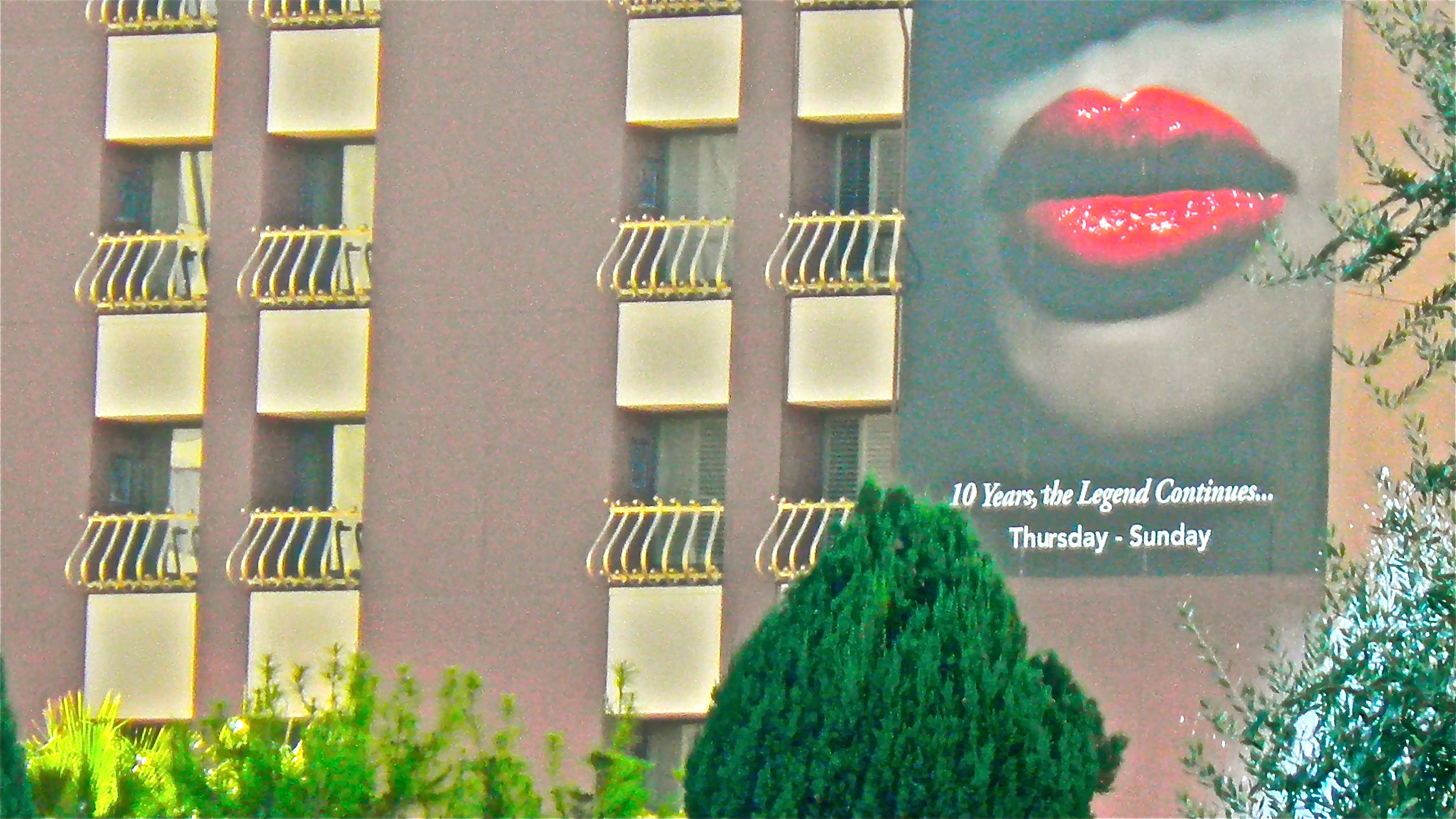The image showcases a large apartment building with numerous windows, each featuring small balconies. In front of the building, there are well-maintained bushes with vibrant green leaves, along with a distinctive evergreen tree that comes to a pointed top. Dominating the side of the building, a striking black poster captures attention. The poster displays a close-up of a woman's face, focusing on her shiny, red lips, which are partially covered by a black line just below her nose. Beneath the image, a bold white caption reads, "10 years, the legend continues Thursday through Sunday." The combination of the apartment building's modern architecture and the eye-catching poster creates a visually appealing and dynamic scene.